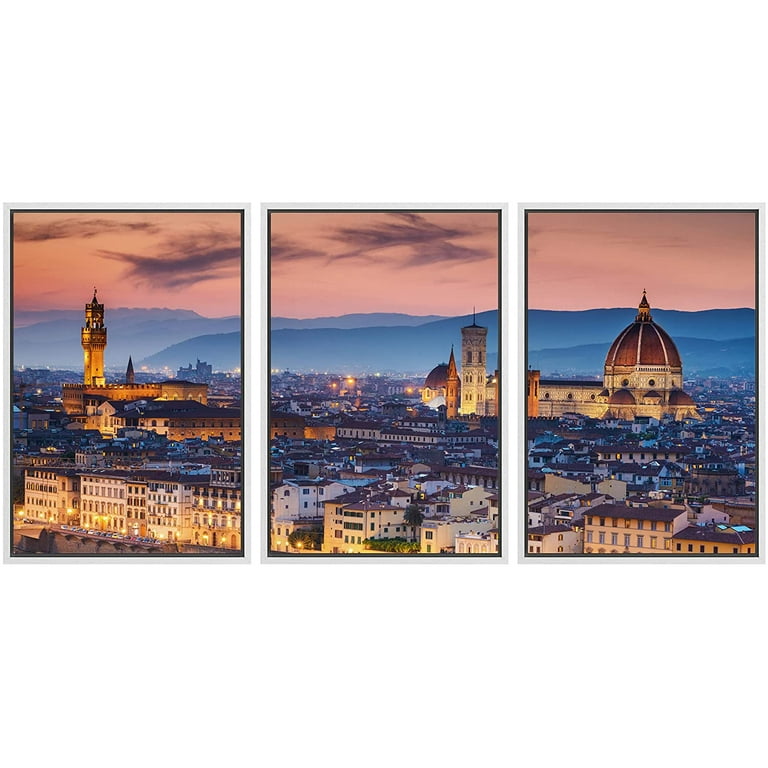The image, framed as three adjoining vertical sections, collectively forms a panoramic view of a European-style city set against a mountainous backdrop with a white sky tinged with hues of orange and pink, suggesting sunrise or sunset. The city's landscape is marked by various beige buildings with burgundy-red rooftops, predominantly three to four stories high, but highlighted by two major structures. On the left, a castle with a prominent square tower is visible. The center and right parts of the image showcase a grand cathedral, its architecture distinguished by several round towers and a large dome on the far right, which stands out with its rich coloration and illumination. The sky above features navy blue mountains and dark clouds. Despite the general dimness, the scene is accentuated by the warm, glowing lights from within the buildings, giving life to the urban expanse below the serene and dramatic skyline.